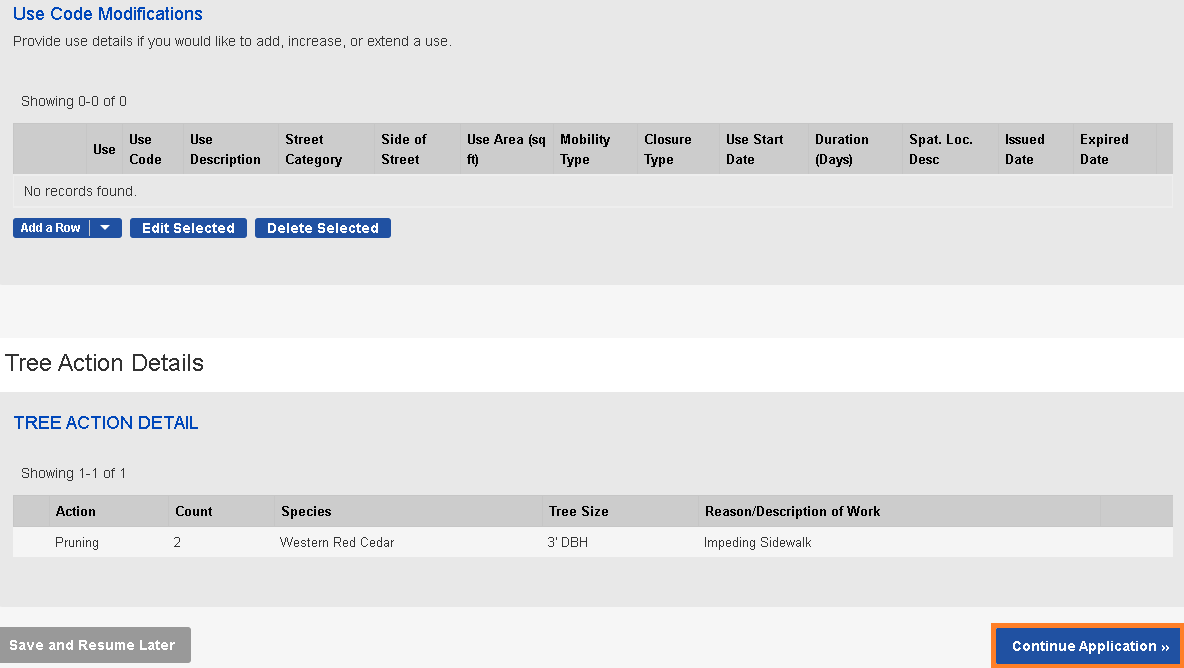**Descriptive Caption:**

The image depicts a detailed data entry page for managing and modifying use codes. At the top, it instructs users to "use code modifications" and underneath, it states in black text, "Provide use details if you would like to add, increase, or extend a use."

The main section of the page features a data row with a message indicating "Showing 0 of 0" and "No records found," accompanied by various categories such as:
- Use
- Use Code
- Use Description
- Street Category
- Side of Street
- Use Area
- Mobility Type
- Closure Type
- Use Start Date
- Duration
- SPAT
- LOKE
- Desk
- Issued Date
- Expired Date

There are blue buttons with white text labeled "Add a Row," "Edit the Selected," and "Delete the Selected."

At the bottom of the page, there is a segment titled "Tree Action Details." It repeats the title "Tree Action Details" in blue and shows data: "Showing 1 of 1" with the action listed as "Pruning," the count as "2," the species as "Western Red Satyr," the tree size as "3 DBH," and the reasons/description of work noted as "Impeding sidewalk."

Additionally, there is a grey button labeled "Save and Resume Later" and a blue button labeled "Continue Application."